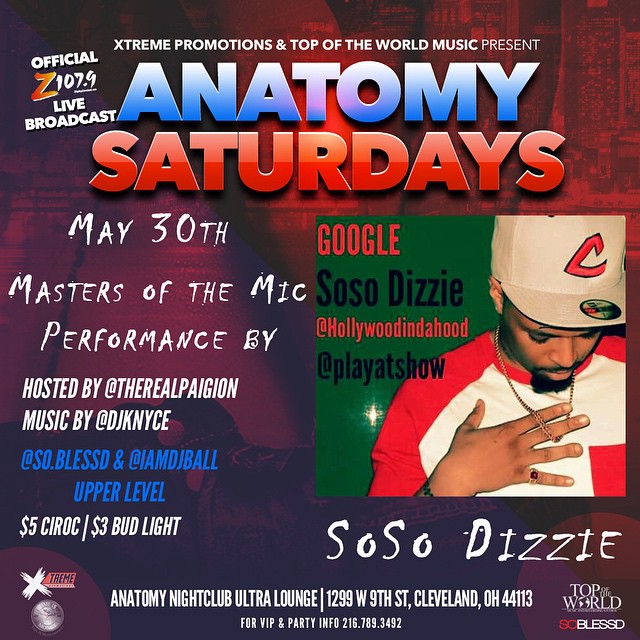**Detailed Event Advertisement Caption:**

Extreme Promotions and Top of the World Music Present: Anatomy

Join us on Saturdays for an electrifying experience at Anatomy Nightclub Ultra Lounge! This official Z 107.9 live broadcast guarantees a night full of fun and excitement. 

Event details:
- **Date:** May 30th
- **Event Title:** Masters of the Mic Performances
- **Host:** @TheRealPagan
- **Music by:** @DJKniez, @SoBlessed, and @IAmDJBall (Upper Level)
- **Special Offers:** $5 Ciroc and $3 Bud Light

The event flyer features an image with a green background of a man in a red and white shirt and a baseball cap with a "C" on it. He sports a gold chain and is captioned, "Google So So Dizzy at Hollywood Indahood at Play At Show." This portrays the featured performer, So So Dizzy.

Venue details:
- **Location:** Anatomy Nightclub Ultra Lounge, 1299 West 9th Street, Cleveland, Ohio 44113
- **Contact for VIP and party info:** 216-789-3492 

Don't miss out on this incredible night of music and performances!